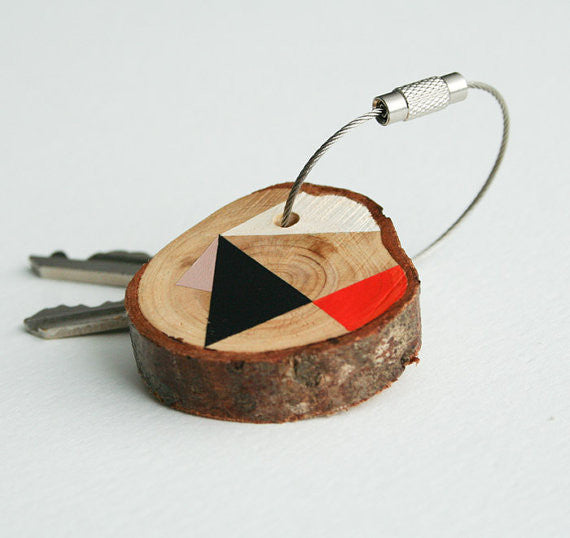The image displays a close-up of a keychain against a white background. The keychain consists of a metallic chain connecting two keys, partially obscured by a circular wooden piece. This piece of wood, likely cut from a thick tree branch, serves as the key holder. It's painted on the top with four distinct geometric shapes: a large black triangle, a medium red triangle, a small pink triangle, and a white triangle. The wood itself features a combination of light and dark brown tones. The metallic chain includes a silver clasp and a small silver pole going through a hole in the wooden key holder, securing the keys. The background is a minimalistic white, emphasizing the details of the keychain and its components.